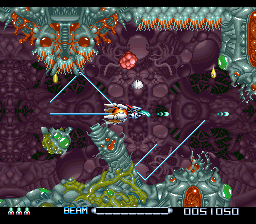The image appears to be a vintage screenshot of an arcade or television video game from the 1980s, characterized by its classic font style reminiscent of that era. The game's interface comprises a maze-like structure with a vibrant purple background, featuring an intriguing pattern that adds visual complexity. At the top, there is a banner with light green and orange elements, possibly signifying a header or title area within the game.

Central to the image is a depiction of a spaceship or astronaut, suggesting an outer space or galaxy-themed adventure. The presence of the word "beam" on the bottom further reinforces the space-related context, indicating a possible in-game mechanic or feature.

The numerical display shows "005" and "1050," which likely represents player scores or game levels. Additionally, three small rocket symbols are positioned on the bottom left, potentially indicating the player's remaining lives or energy within the game.

Overall, the image captures the essence of retro gaming with its distinct visual and thematic elements, evoking a sense of nostalgia for classic sci-fi arcade adventures.